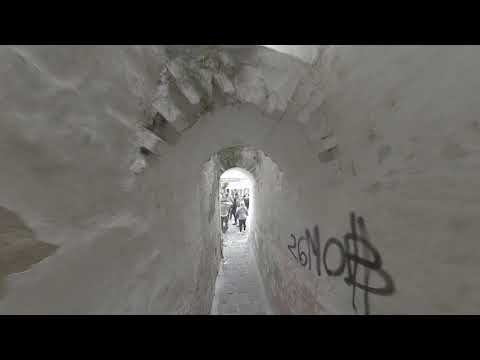The image depicts a long, narrow, and almost entirely white tunnel-like alleyway, framed by textured stone or stucco walls exhibiting signs of wear and erosion. The walls display graffiti that reads "26MOB," with the 'B' distinctly marked by two vertical strikes, suggesting a dollar sign. Towards the far end of this covered walkway, there is a brighter area illuminating a distant group of people clad in hooded sweatshirts, making it hard to discern their activities. The texture of the tunnel is varied, with dingy areas, particularly noticeable on the upper left of the archway, possibly from mildew or smoke stains. The image has a black border on the top and bottom, giving it the appearance of a black and white photograph.